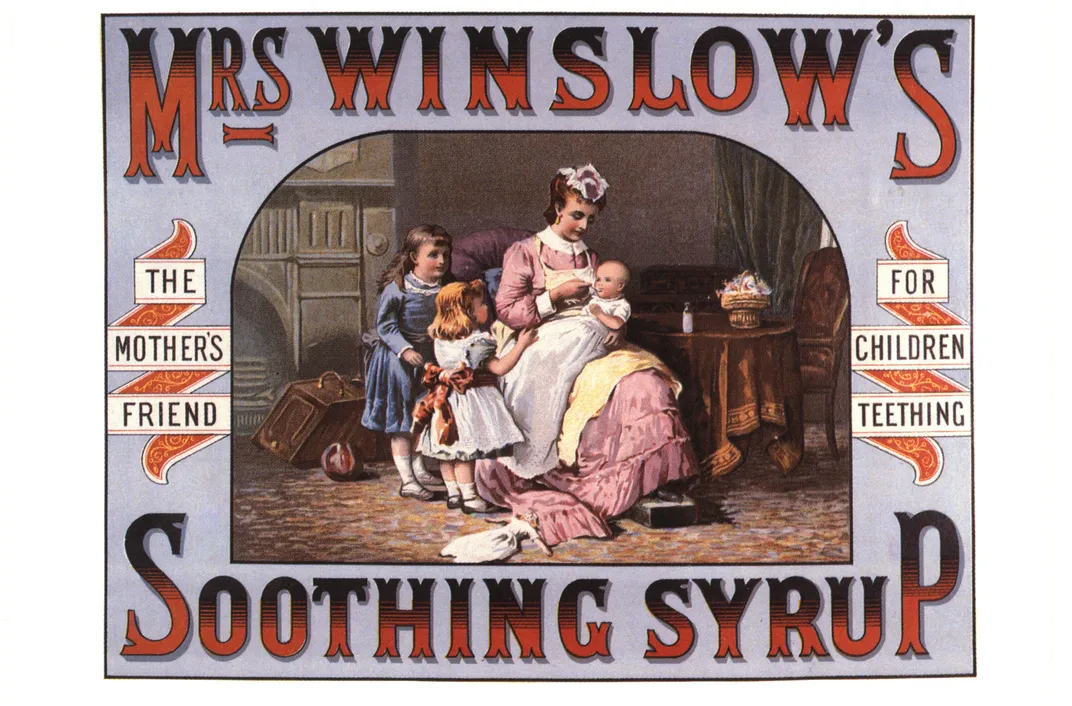The advertisement is a nostalgic piece from the 1800s or early 1900s, featuring a richly illustrated scene framed by a blue border. The top of the advertisement prominently displays the brand name "Mrs. Winslow's," with letters that transition from black at the top to a medium shade of brown. Below the central image, the purpose of the product is clearly stated: "soothing syrup." On the left, a small banner reads "the mother's friend," while the right side declares "for children teething," both in black letters against a white background.

The central image depicts an elegantly dressed woman seated in a purple chair, wearing a long-sleeved, elaborate pink dress with an apron. She tenderly offers a spoonful of syrup to the baby on her lap, who is dressed in a long white gown. Two other children stand beside her, one in a blue dress and the other in a white dress. The background includes various household items: a round table with a brown covering, possibly holding a small bottle of milk and an arrangement, a chair, a green drapery, a suitcase, and a ball on the floor.

The detailed illustration captures a serene, nurturing moment, highlighting the product's promise to soothe teething children and be a dependable aid for mothers.